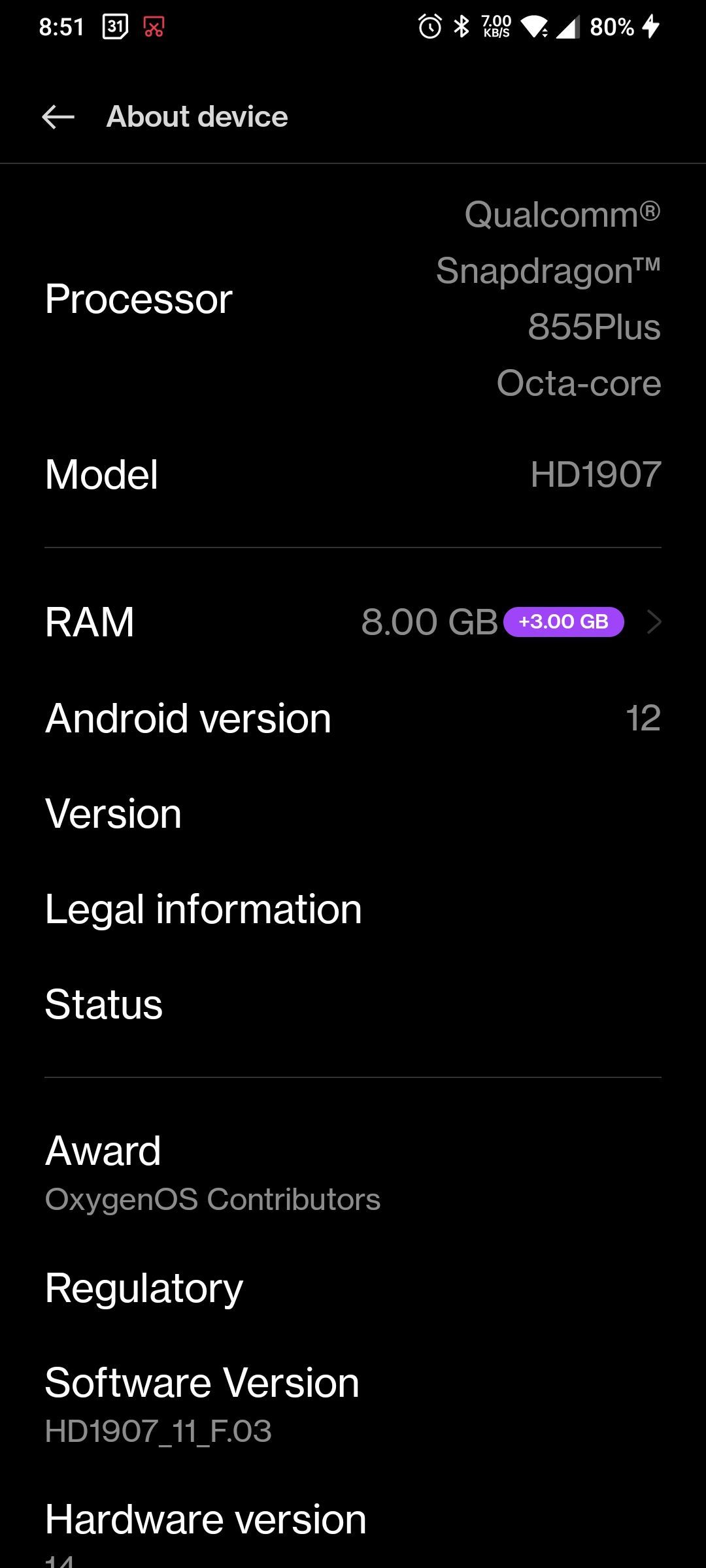This is a vertical mobile screenshot with a black background. 

- Top-left corner: Battery icon and "8:51"
- Top-right corner: Battery percentage at "80%".
  
### Main content:
- **Header**: "About Device" with a back arrow.
- **Processor Information**: "Qualcomm Snapdragon 855 Plus, Octa-core".
- **Model Number**: "HD1907".
  
### Dividing Line
- **Horizontal gray line** 
  
### Memory Information:
- **RAM**: "8 GB" with a note "Plus 3 GB" in purple.
- **Android Version**: "12".
  
### Additional Menu Items:
  - "Version"
  - "Legal Information"
  - "Status"
  
### Dividing Line
- **Horizontal gray line** 
  
### Extra Information:
- **OxygenOS Contributors**
- **Regulatory Information**
- **Software Version**: "HD1907_11_F.03"
  
### Footer:
- **Hardware Version**